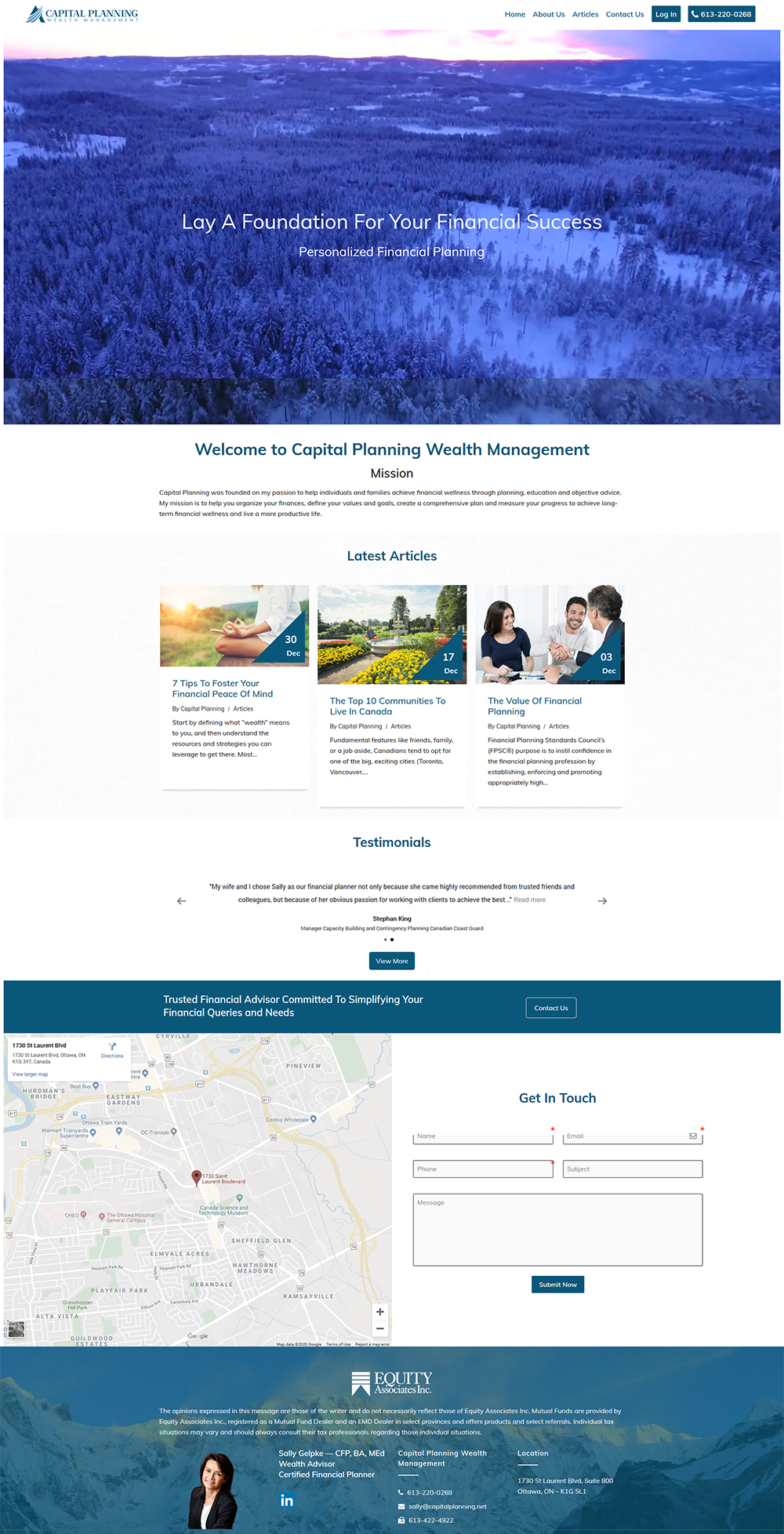The website features a well-organized layout with distinct sections for easy navigation. At the top left corner, in blue text, it reads "Capital Planning" followed by "Wealth Management". On the top right side, there are clickable buttons labeled "Home", "About Us", "Articles", "Contact Us", a dark blue "Login" button in white text, and a button displaying the telephone number (613-222-220-0268) in white along with a phone icon.

The background features a scenic image of a sky transitioning from white to shades of purple and violet, overlaying a landscape with gray mounds and green trees illuminated by a blue hue. Centered in white text, it highlights the slogan "Lay a foundation for your financial success" with the subtitle "Personalized Financial Planning" beneath it. Surrounding these elements is a welcoming message in dark blue text: "Welcome to Capital Planning, Wealth Management".

Below this central section, the website showcases "Our Mission" in black text, detailing the company's objectives. The "Latest Articles" section follows, featuring an image of a person meditating in a white shirt facing a forest, dated September 30th or December 30th. The accompanying article title in bold blue reads, "7 Tips to Foster Your Financial Peace of Mind". 

A subsequent article titled "The Top 10 Communities to Live in Canada", dated December 17th, is introduced with an image of a garden with yellow flowers, green plants, green trees, and a partly cloudy blue sky.

In the "Testimonials" section, an image shows a group of people conversing around a table. A woman in a dark blue dress with short black hair is smiling, alongside a man in a gray long-sleeved shirt with a white undershirt, black hair, and a short mustache who is also smiling and shaking hands. Additionally, an older individual with hair transitioning from brown to black to gray, dressed in a black suit with a white dress shirt, is depicted shaking hands. This section describes a testimonial with the text: "My wife and I chose Sally as our financial planner not only because she came highly recommended from trusted friends and colleagues but because of her obvious passion for working with clients to achieve the best". Below that, in gray text, it reads "Read More", and the testimonial is attributed to "Stephen King" in bold black text, listed as "Manager Capacity Building and Contingency Planning".

At the bottom of the page, a map is displayed, followed by the company's contact information.